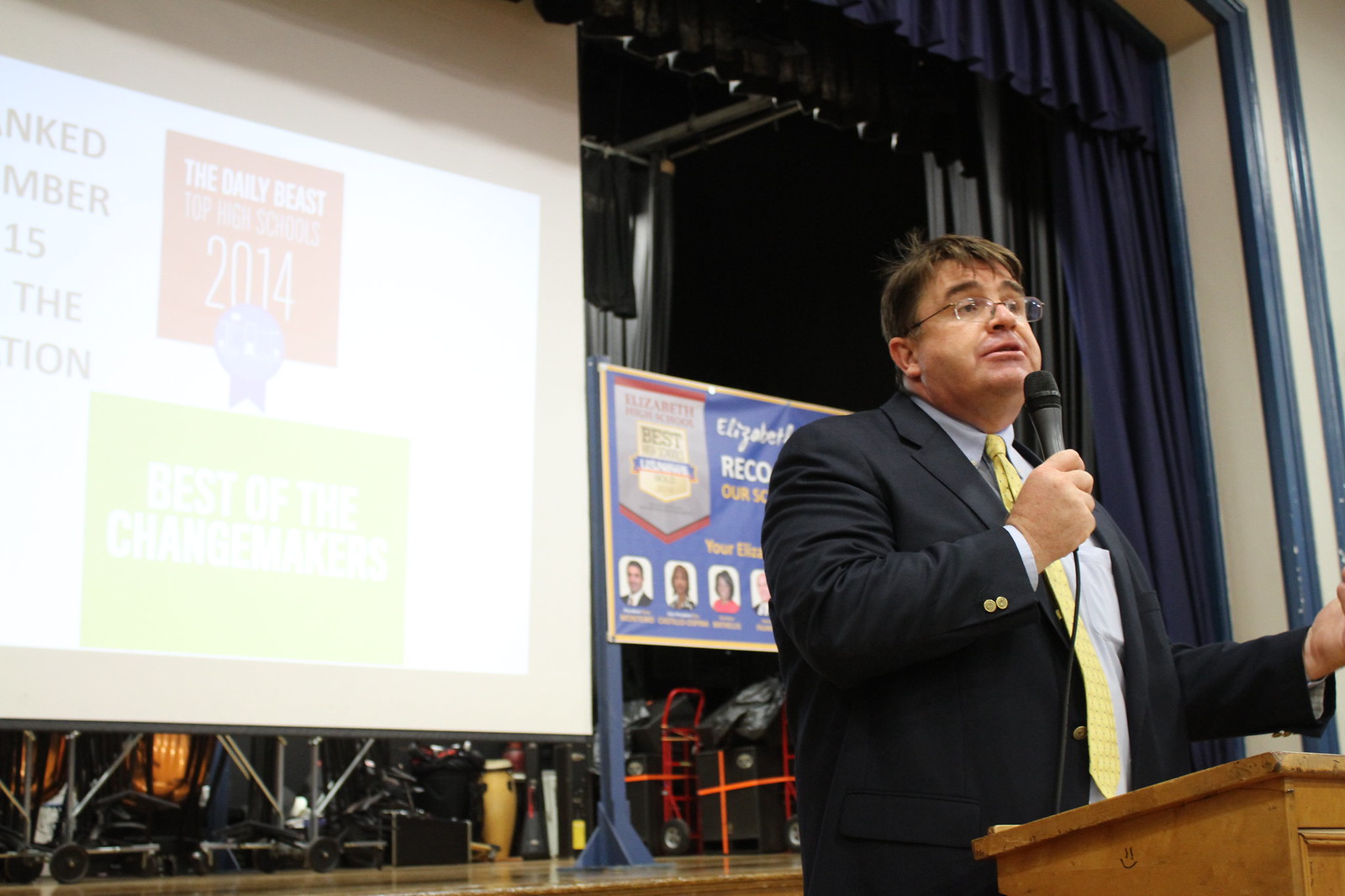The image captures an older, slightly heavier set Caucasian man with short brown hair and glasses, standing confidently at a brown wooden podium adorned with a small smiley face. He is dressed in a dark suit with a blue dress shirt and a yellow tie. The man holds a wired microphone in his right hand, which he brings close to his face while his left hand is gesturing upwards. Behind him, a large stage is in clean-up mode, featuring several garbage bins on lifts and scattered metal scaffolding. The backdrop consists of blue curtains and a prominent blue banner displaying indistinct images of people. A massive white projection screen dominates the scene, bearing an image with partially visible text that includes phrases like "the Daily Beast 2014" and "Best of the Changemakers." Bright lights illuminate the indoor setting, highlighting the vibrant yet busy atmosphere of an event winding down.